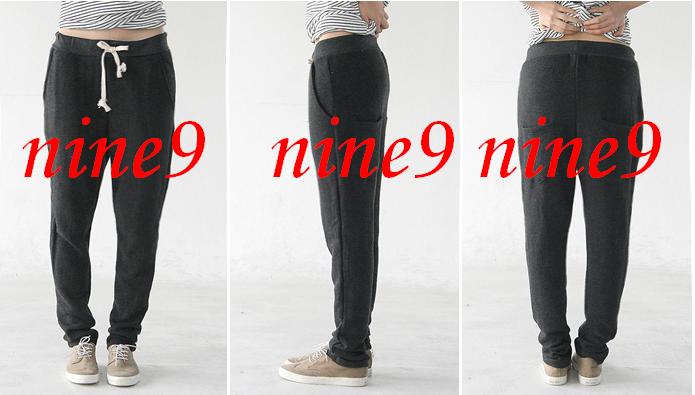This advertisement showcases a set of three photographs arranged horizontally, each presenting a waist-down view of the same model from different angles: front, side, and back. The model is attired in gray sweatpants with a white drawstring and light tan shoes featuring white laces and rubber soles. She pairs the pants with a black and white striped shirt, partially pulled up to reveal a sliver of midriff. Each segment of the triptych highlights a different perspective of the outfit, and a bright red caption reading "nine 9" (with the first 'nine' spelled out and the second in numeral form) spans across all three images. The photographs are framed against a gray background with white dividers, accentuating the clean layout of the advertisement.